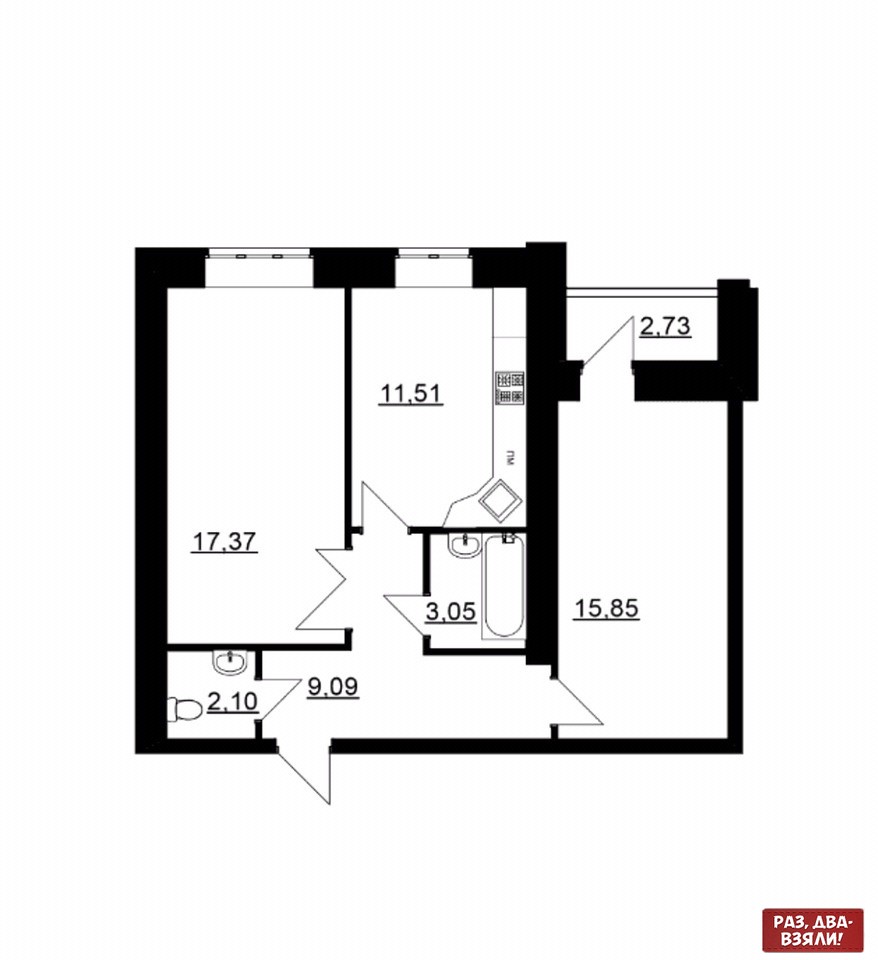This image showcases a detailed floor plan for a section of a home, with all room labels omitted. Noteworthy features and elements are as follows:

- **Lower Right Corner**: A brown rectangle inscribed with white text displays an assortment of characters, "PA3, ABA-B3," and various symbols including a backwards "R," an upside-down "V," a backwards "N," and an exclamation point, hinting at a language or code unfamiliar to the viewer.
- **Walls**: The boundaries of the rooms are denoted by thick black lines, providing a clear demarcation of spaces within the floor plan. 
- **Rooms**: 
  - **Room 1**: 
    - On the right side, a space potentially designated as a porch due to its positioning and lack of specified features.
  - **Room 2** (Kitchen): 
    - Contains typical kitchen fixtures.
  - **Room 3** (Bathroom): 
    - Equipped with a sink and a bathtub.
  - **Room 4** (Half-Bath): 
    - Includes a sink and a toilet.
- **Hallway**: 
  - An upside-down T-shaped corridor connects several rooms, facilitating movement throughout the home.
- **Measurements**: 
  - Numbers are present, though there are no units to clarify the dimensions they represent.
- **Windows**: 
  - The house appears to feature only two exterior windows, limiting natural light and vistas.

This comprehensive description highlights all observable elements, presenting an accurate and articulate depiction of the floor plan.